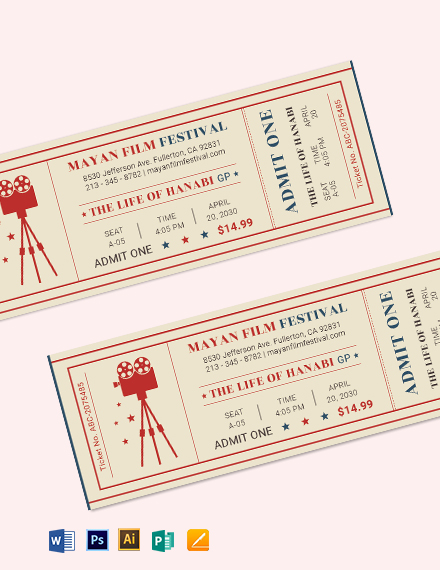The image features two identical tickets to the Mayan Film Festival, displayed at a slight angle ascending to the right, set against a light pink background. Each ticket has a tan backdrop and prominently features an illustration of a red vintage film projector with two spools on the left side. Central to the ticket in bold red and blue text are the event details: "Mayan Film Festival" followed by "8530 Jefferson Avenue, Fullerton, California, 92831," along with a contact number "213-345-8782" and a URL "MayanFilmFestival.com". The main feature film is "The Life of Hanabi," denoted in red. Additional details include "Seat: A-05," "Time: 4:05 PM," "Admit One," and the price "$14.99." The ticket also mentions "April 2023" and a unique ticket number "ABC2075485," alongside an "Admit 1" stub on the right side decorated with a blue text. The color scheme primarily incorporates shades of tan, red, blue, and pink, and the clarity of the tickets suggests a digital creation rather than a photograph, evidenced by photo editing indicators below the tickets.